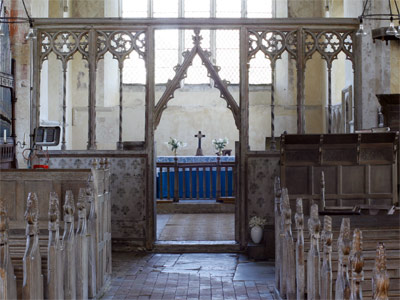The image depicts the interior of a very old Catholic church, possibly a chapel within a larger cathedral. The scene is viewed from the middle of the aisle, flanked by rows of long wooden pews on either side. At the focal point of the image is an ornate archway with a triangular top, featuring panel barriers and cutout spaces that provide a view into the altar space beyond. The archway is adorned with intricate carvings that might be wood or stone, adding to the sense of antiquity and reverence. 

Beyond the archway, the altar is draped with a dual-layered tablecloth, the top one being light blue over a darker blue. Flanking the central cross or crucifix on the altar are two bouquets of white flowers, enhancing the sacred ambiance. The background is illuminated by tall, bright windows, which let natural light pour into the space, casting a serene glow on the yellow-white walls. The floor appears to be made of old bricks, contributing to the historical atmosphere of the church. The image captures a moment of empty tranquility, devoid of any congregants, highlighting the church's grandeur and timeless beauty.